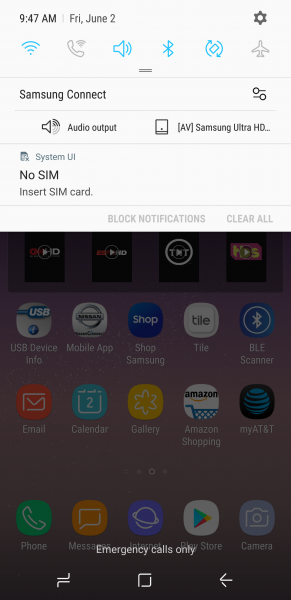The image showcases a cell phone screen with various interface details and notifications. At the top left corner, it displays the current time, 9:47 a.m., along with the date, Friday, June 2. On the top right corner, there is a gear icon indicating settings. Directly below these icons are multiple status symbols: a wireless signal, a phone logo, a speaker icon, a Bluetooth symbol, two circular arrows, and an airplane icon, likely indicating various connectivity statuses and the phone being in airplane mode.

Beneath these icons, the text "Samsung Connect" appears prominently. Below this text is a microphone icon accompanied by the words "Audio Output." There is then a notification stating "No SIM - Insert SIM card," indicative of a missing SIM card. Further down, the options "Block notifications" and "Clear all" are displayed.

The majority of the screen is taken up by an app menu, which is darkly overlaid, making it difficult to discern specific icons clearly. Nevertheless, apps and their names are visible, including USB Device Info, Mobile App, Shop Samsung, Tile, BLE Scanner, Email, Calendar, Gallery, Amazon Shopping, and My AT&T.

At the bottom of the screen, there are additional app icons: Phone, Messages, Internet, Play Store, and Camera. Notably, in white text at the very bottom of the screen, it reads "Emergency calls only," indicating the phone is not fully connected to a network.